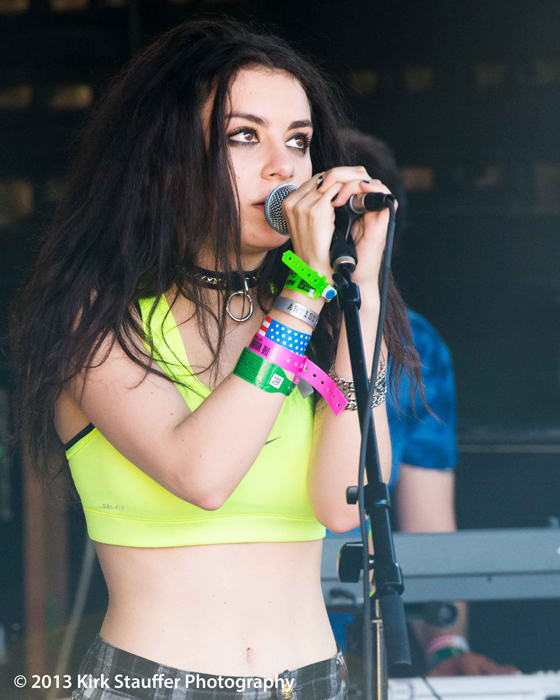This is a detailed photograph capturing Charli XCX in mid-performance on stage. She is wearing a lime green sports bra and what looks like plaid shorts or a skirt, revealing her midriff. Her hair, a dark brown shade, cascades past her shoulders with a slightly unkempt, wavy texture. Charli's eyes are accentuated with heavy black eyeliner and dark eyeshadow. She has multiple wristbands on her left wrist - including lime green, gray, magenta, and American flag designs - and a chain bangle on her right wrist. Her neck sports a black choker with a silver ring dangling from it. She grips the black microphone with both hands, showcasing her black nail polish. Behind her, a man in a blue shirt is playing an electric keyboard. The stage backdrop is dark with lights scattered around it. In the bottom left corner of the photo, a copyright mark reads, "2013 Kirk Stoffer Photography.”